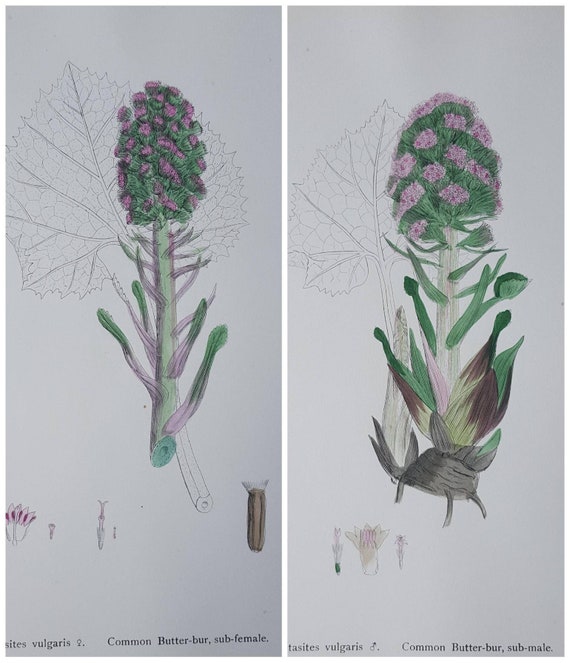The image showcases two detailed botanical sketches of the Common Butterbur plant, each representing a different sex. The drawings are presented side by side on a vertically oriented off-white or very light gray background. Both halves of the image highlight the intricate structure of the plant, with colored illustrations superimposed on a black and white ink or pencil drawing of a large leaf in the background.

On the left-hand side, the Common Butterbur Subfemale is depicted. This sketch features a cylindrical green stem with green and purple leaves extending from the lower half. The top part of the stem displays green needle-like structures adorned with small, unopened purple flowers. The text at the bottom reads "Common Butterbur Subfemale."

Conversely, the right-hand side illustrates the Common Butterbur Submale. Similar in overall structure, this sketch shows the flowers in a lighter purple hue and more fully bloomed compared to the Subfemale. Additionally, there are larger leaves at the base of the stem. The Submale's base integrates into a larger brown root structure, and the branches off the stem are darker green. The text at the bottom here reads "Common Butterbur Submale."

Both sketches also include the species name "something vulgaris" followed by the respective gender symbols, providing a scientific and artistic representation of the male and female varieties of the Common Butterbur.